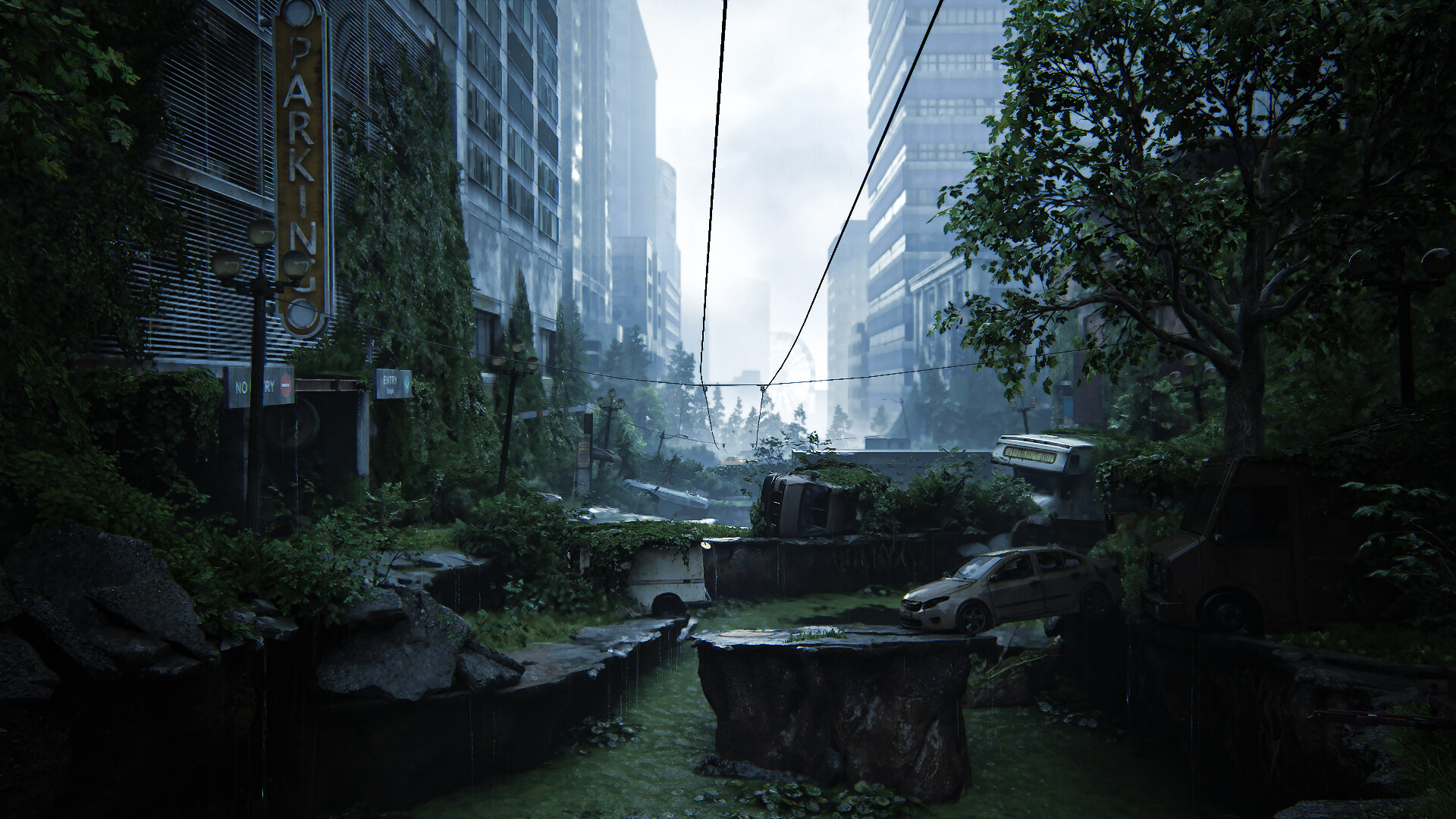**Detailed Caption:**

The image depicts a beautifully detailed, post-apocalyptic cityscape, likely from a video game or concept art. The scene captures an abandoned urban environment that has been reclaimed by nature. A cracked and overgrown street runs vertically from the bottom center to the midpoint of the image, guiding the viewer’s eye towards the vanishing point. Flanking the street on both sides are towering, dilapidated buildings, possibly remnants of apartment complexes or business structures, emphasizing the height and scale of the city. Central to the scene, above the horizon and near the exact middle of the image, is a small, bright window. This window frames a hazy, white sky partially obscured by drifting smoke, adding an atmospheric touch to the desolate yet striking tableau.